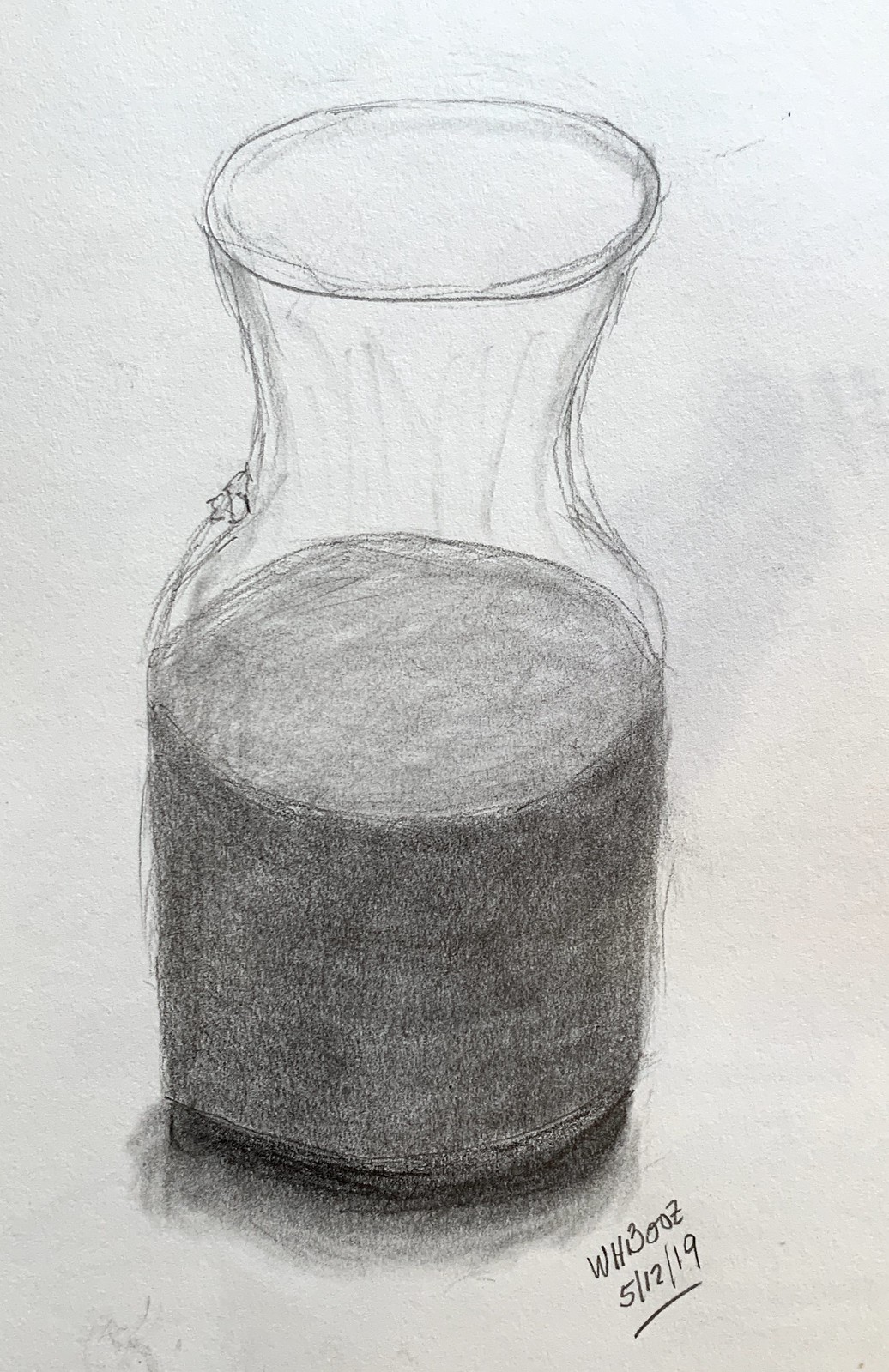This detailed charcoal sketch on white drawing paper depicts a glass flask with an intricate structure and thoughtful shading to create a realistic three-dimensional effect. The flask features a cylindrical base that gently narrows before flaring out again towards a slightly circular bottom. It has a ribbed texture at the top, marked by precise pencil lines, and a tapering neck forming a cone shape. Approximately 60% of the flask is filled with a dark gray liquid, which deepens to an almost black hue at the bottom, indicating a shadow rather than the actual liquid level. This dark portion is highlighted by lighter gray shading that extends in front, enhancing the three-dimensional illusion. There may be subtle etchings on the neck of the flask, potentially hinting at a floral design. The drawing is signed "WHI300Z" with a line through the "Z" and dated "5/12/19" with a line underneath in the bottom right corner, adding a personal touch by the artist.